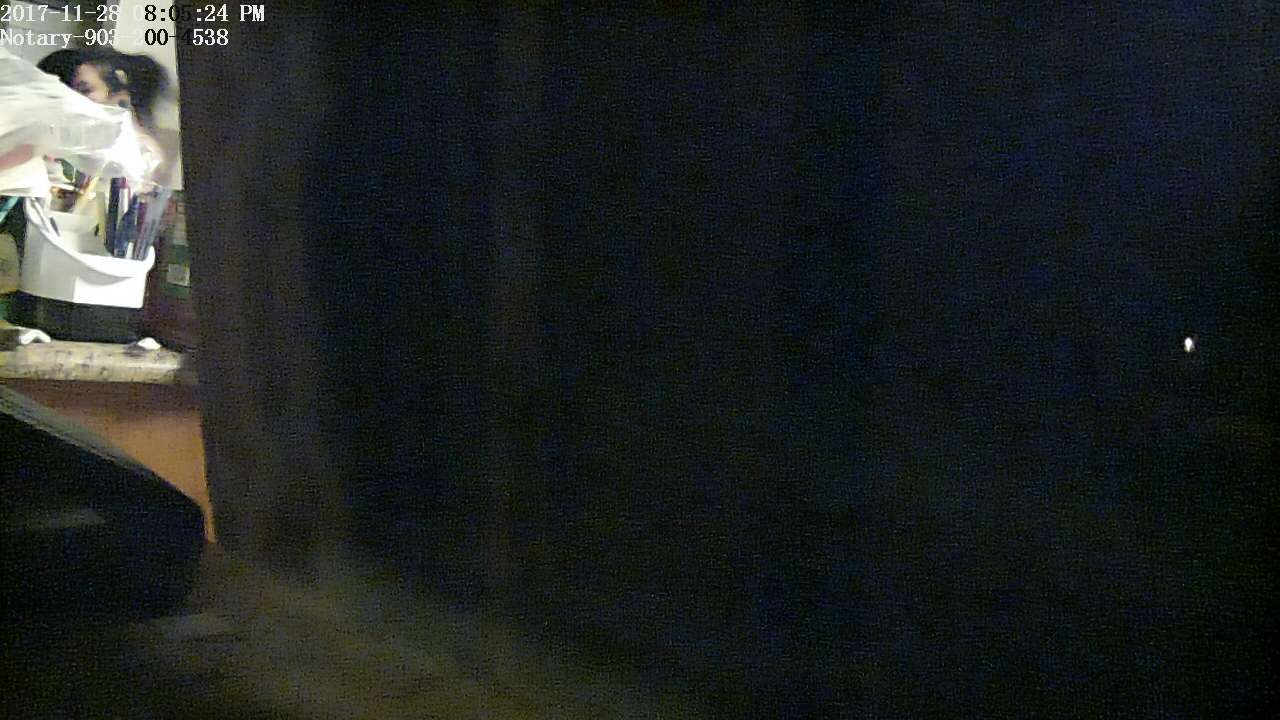In a dimly lit room with a partially open door, only a small section on the left side of the image is illuminated. The scene appears to be set in a hair salon. A person is seated behind a tan cabinet with a marble top, with a white device resembling a set of curlers placed on the table. The cabinet is covered with a plastic drop cloth, but the white device remains exposed. The individual in the picture has large earrings and their hair seems to be in the process of being styled. The timestamp on the image reads November 28, 2017.